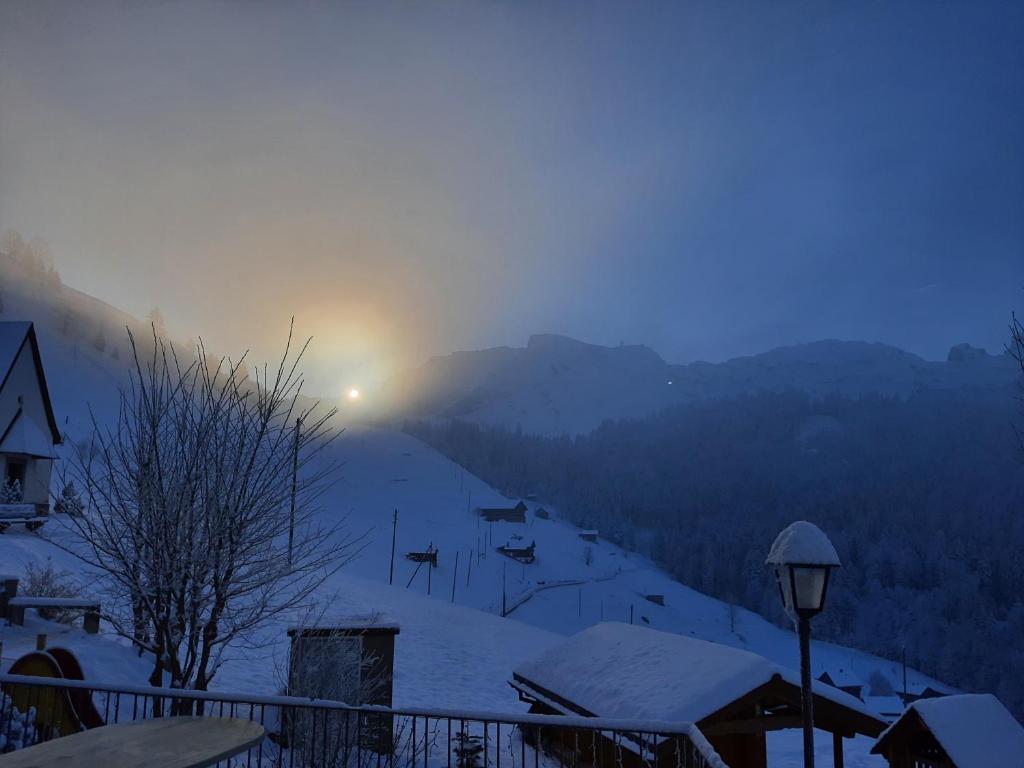The photograph captures a tranquil, snowy landscape at dawn. In the foreground, a snow-covered street lamp and a metal fence stand prominently against the serene, light blue backdrop of the town. Sparse, barren trees and rooftops dusted with snow add to the quiet stillness. The slope of the hillside starts from the upper left corner, descending toward the bottom right, dotted with a few buildings that emerge from the blanket of snow. In the distance, blue-outlined mountains form a majestic backdrop. The sky, transitioning from the dark hues of night, boasts a faint rainbow effect as the sun peeks over the mountains, casting a gentle orangey-yellow glow that hints at the arrival of a new day.